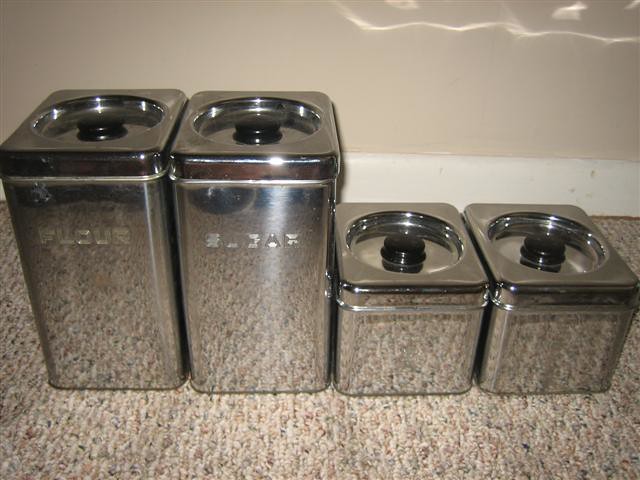The photograph depicts four metallic canisters with a silver finish, positioned against a cream-colored wall with a white skirting board at the bottom. The canisters are placed on a textured carpet that has a mix of brown tones and some light and dark stony patterns, mimicking the look of brick flooring. The two canisters on the left are tall and rectangular, while the two on the right are shorter and cubic, approximately half the height of the tall ones. The canister on the far left has the word "flour" etched into its surface, and the one next to it is labeled "sugar". Both labels are etched into the metal, allowing the reflective surface to show the carpet's pattern through them. The two smaller canisters on the right are unlabeled. All four canisters feature square tops with a circular indentation and a black knob in the center.